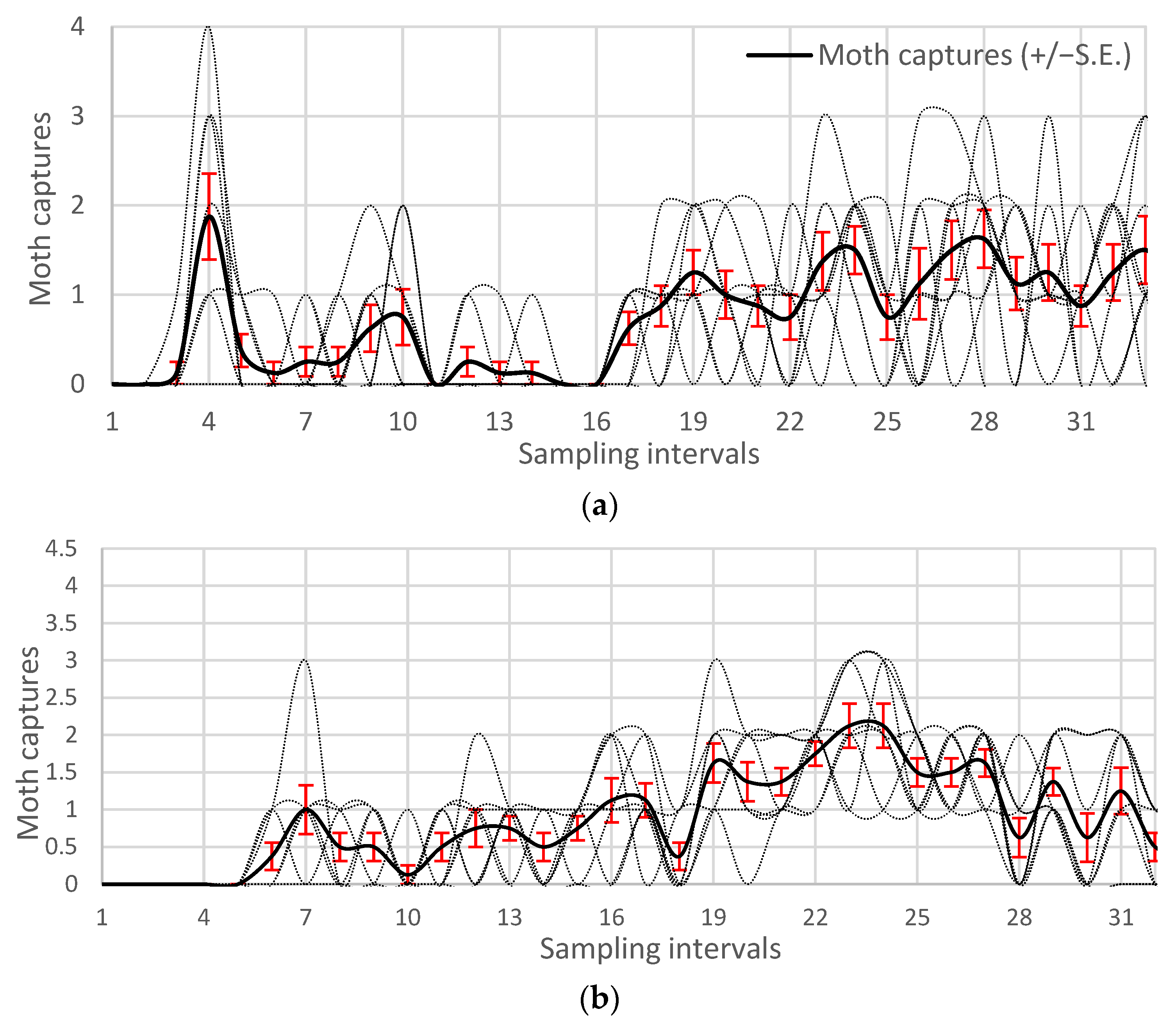This image consists of two vertically stacked graphs labeled A and B, both depicting moth captures. The y-axis of the top graph (A) is labeled "Moth Captures" and ranges from 0 to 4 in increments of 1, while the bottom graph (B) ranges from 0 to 4.5 in increments of 0.5. The x-axis on both graphs is labeled "Sampling Intervals" and spans from 1 to 31, with intervals numbered by each day. A key in the top right corner of each graph explains that the solid black lines denote "Moth Captures (±S.E.)". The graphs showcase a series of wavy parabolic curves in black and gray, with interspersed red bars marked with letters "I". These curves rise and fall, tracking the moth captures over time, and are visually similar between the two graphs, illustrating the moth population fluctuations at different sampling intervals.